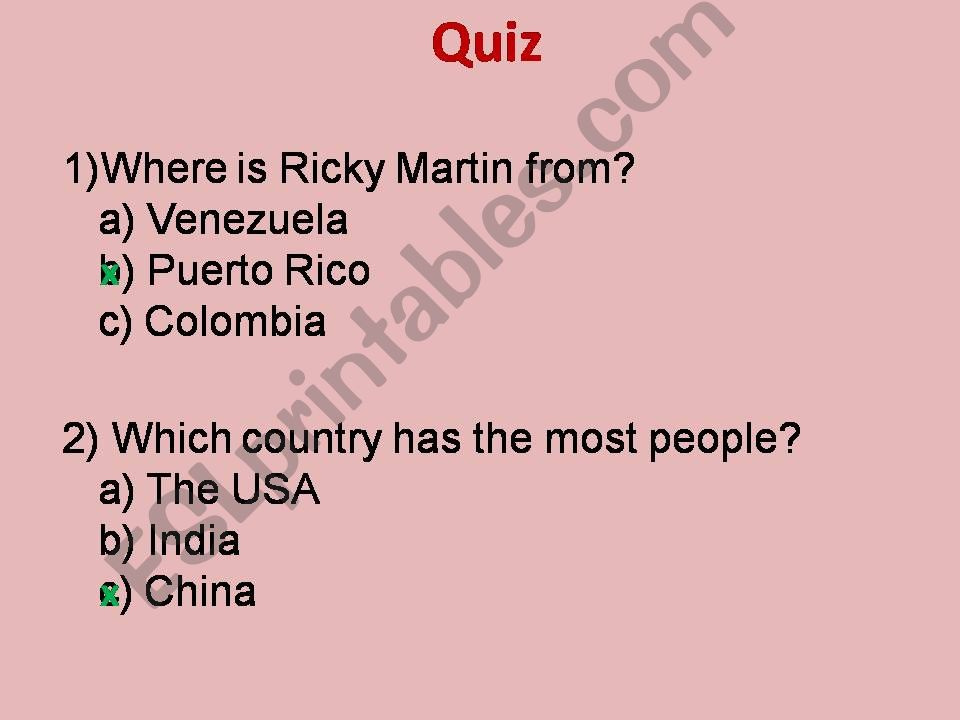The image is a screenshot of a light pink background with text overlay featuring a simple online quiz. The text is handwritten and somewhat uneven. At the top center, the word "Quiz" is presented in red. Below it are two multiple-choice questions. 

1. "Where is Ricky Martin from?" 
   - A) Venezuela
   - B) Puerto Rico (marked with a green X)
   - C) Colombia

2. "Which country has the most people?"
   - A) The USA
   - B) India
   - C) China (marked with a green X)

Diagonally spanning from the lower left to the upper right of the image, there is a noticeable watermark in large gray text that reads "ESLPrintables.com." The overall aspect ratio of the image appears to be approximately 4:3.

The presence of the watermark and the simple nature of the quiz hint that the content may have been sourced from an educational material website.